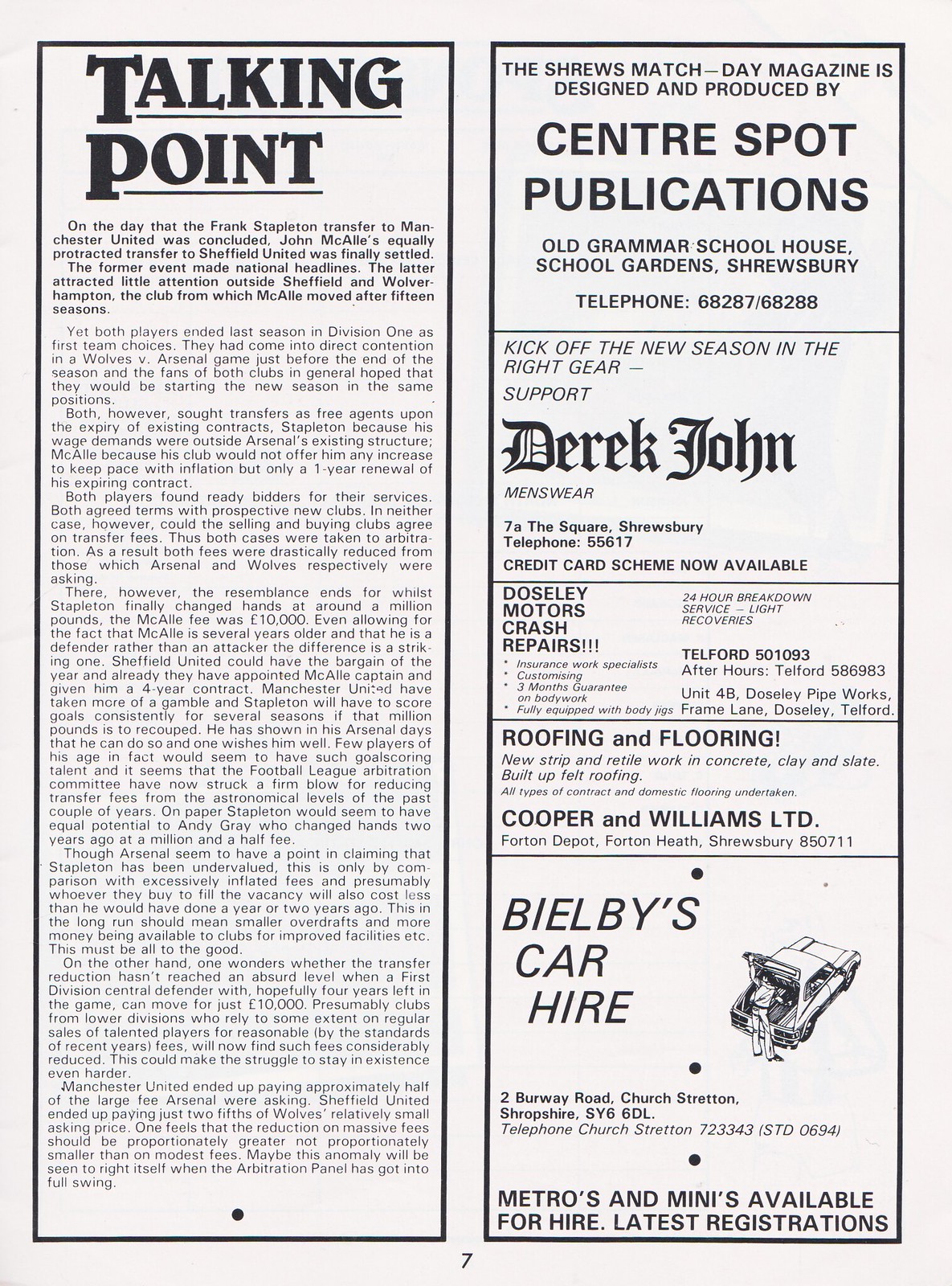This black and white newspaper clipping from "The Talking Point" is printed on white cardstock and bordered with black. Dominating the left side in bold black type is the newspaper's title, "Talking Point." The article covers the conclusion of two significant football player transfers: Frank Stapleman's move to Manchester United, which made national headlines, and John McAley's transfer to Sheffield United from Wolverhampton after 15 seasons, which garnered little attention outside Sheffield.

The bottom left corner of the page is marked with the number 7, indicating its position within the newspaper. On the right side, there are several advertisements, each accompanied by telephone numbers. Ads feature Derek John Menswear encouraging readers to "Kick off the new season in the right gear," as well as promotions for Doseley Motor Crash Repairs, Cooper and Williams Roofing and Flooring, Blobley's Car Hire, and Bilby's Car Care. Additionally, there is a note that the Shrews Match Day Magazine is designed and produced by Centerspot Publications based at the Old Grammar School House in Shrewbury.